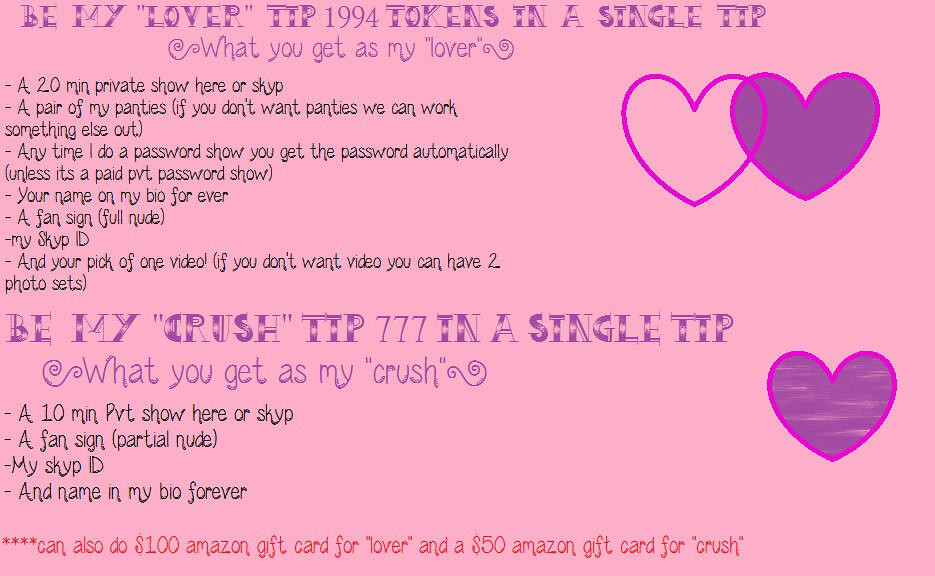The image is a digital card with a predominantly pink background, blending color illustration, typography, and graphic design in a landscape orientation. The right side features three hearts: the top heart is outlined in a purplish shade, the middle heart is filled with a purple hue, and the bottom heart is highlighted with a pinkish-purple outline containing a textured purple fill. The text on the card is a mix of black, purple, and red. 

At the top, decorative purple text announces, "Be My Lover, Tip 1994 Tokens in a Single Tip." Below, it details in black text the benefits of such a tip: "A 20 minute private show here or on Skype, a pair of my panties (or an alternative if declined), automatic password access unless it’s a paid private show, your name in my bio forever, a fan sign, full nude access, my Skype ID, and your choice of one video or two photo sets."

Further down, a subheading in deep pink reads, "Be My Crush, Tip 777 in a Single Tip," followed by: "10 minute private show here or Skype, a fan sign, partial nude, my Skype ID, and your name in my bio forever."

At the bottom, in red text and marked with asterisks, it offers a transactional option: "$100 Amazon gift card for 'lover' and a $50 Amazon gift card for 'crush'." The card gives an impression of being an invite or promotional material from a content creator, laying out benefits for different tiers of support.